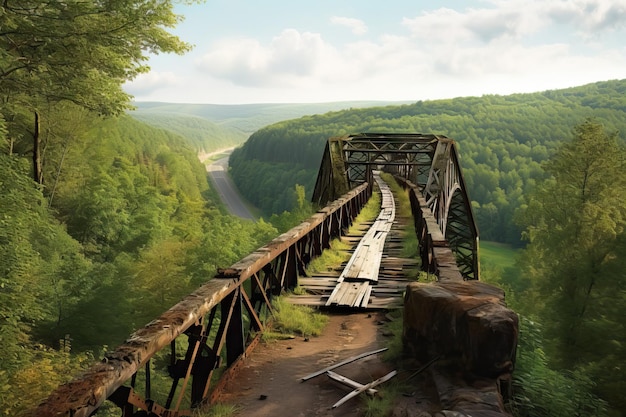This photograph captures an old, abandoned bridge that has clearly seen better days. The bridge, constructed from rusted metal and dilapidated wood, stretches from the foreground to the middle of the image, where it narrows and fades out of focus. A central aisle, once meant for railroad tracks or possibly a walkway, is now overgrown with grass and moss. The entire structure is characterized by extensive rust, with moss adding to its weathered appearance.

Surrounding the bridge is a lush green forest, dominated by dense vegetation and treetops on both sides. Off to the left, a winding road snakes through this verdant setting, flanked by cliffs that create a valley-like impression. The road, situated much lower than the bridge, appears distantly in the background. Above, a light blue sky adorned with white clouds forms a serene backdrop, contrasting with the ruggedness of the bridge. The image's vivid details and realistic yet slightly stylized look give it an almost picturesque or video game-like quality.